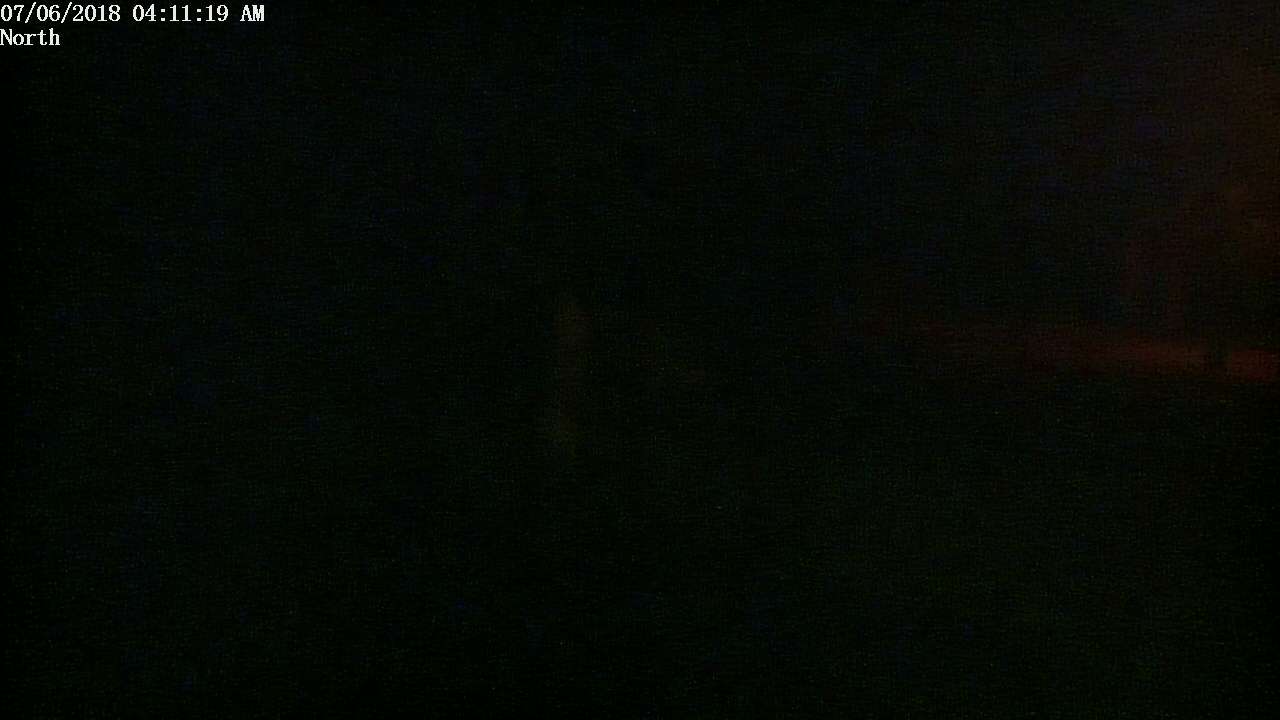The image is a simple, rectangular photograph taken in the dark. The aspect ratio is slightly more than twice as wide as it is tall. The screen or monitor is entirely black except for a small section in the upper left-hand corner. In this corner, white digital text displays the date "07/06/2018" and the time "04:11:19 AM." Directly below this timestamp, the word "North" is written in capital letters. Notably, there is a barely visible brown line running vertically along the extreme right edge of the image, but other than that, the photograph is pitch black. The image likely depicts a moment in the early morning hours of July 6, 2018, oriented toward the north.